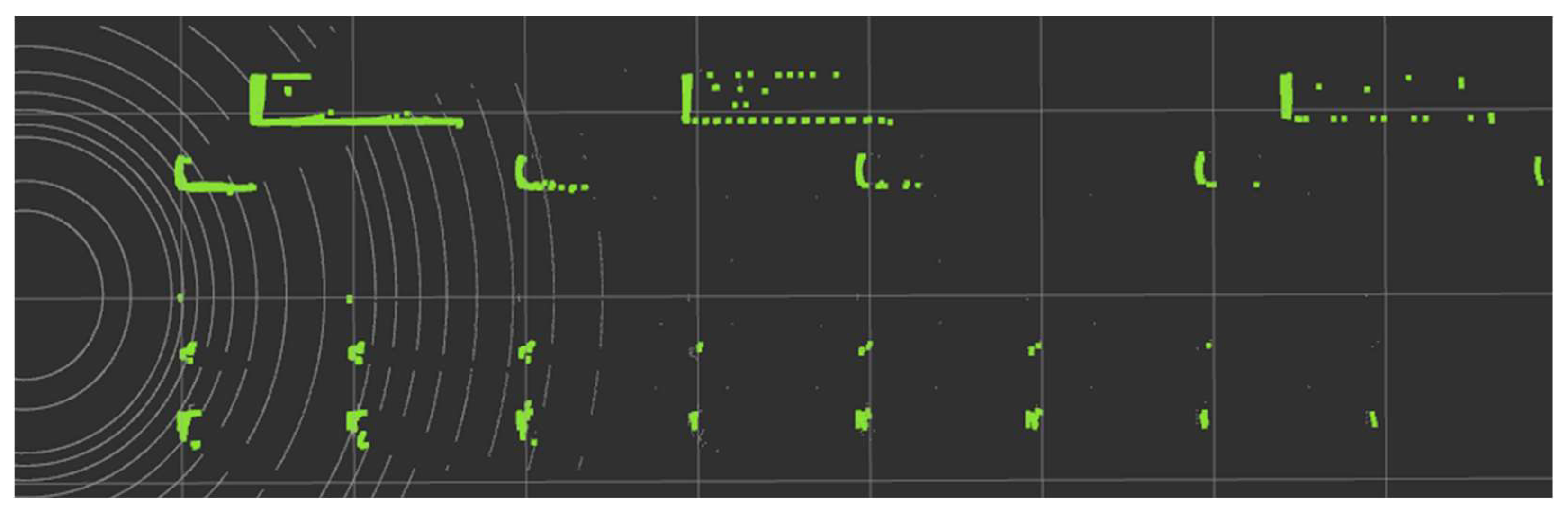The image depicts a rectangular radar screen commonly seen in airports, characterized by a black background and overlaid with a white grid of evenly spaced squares. On the left side of the screen, a series of white concentric circles emanate from a point, extending almost halfway across the image. Scattered irregularly across the screen are bright green spots, some large and some small, which suggest radar blips. These green spots vary in shape and size, with a notable pattern of two rows near the bottom, comprising seven dots on the top row and eight on the bottom row, becoming larger towards the left. The top section of the screen features three distinct larger green lines: one solid, one dotted, and one less dotted. These linear shapes and clusters of green spots convey a detailed radar display, accented against the stark white grid and dark background.